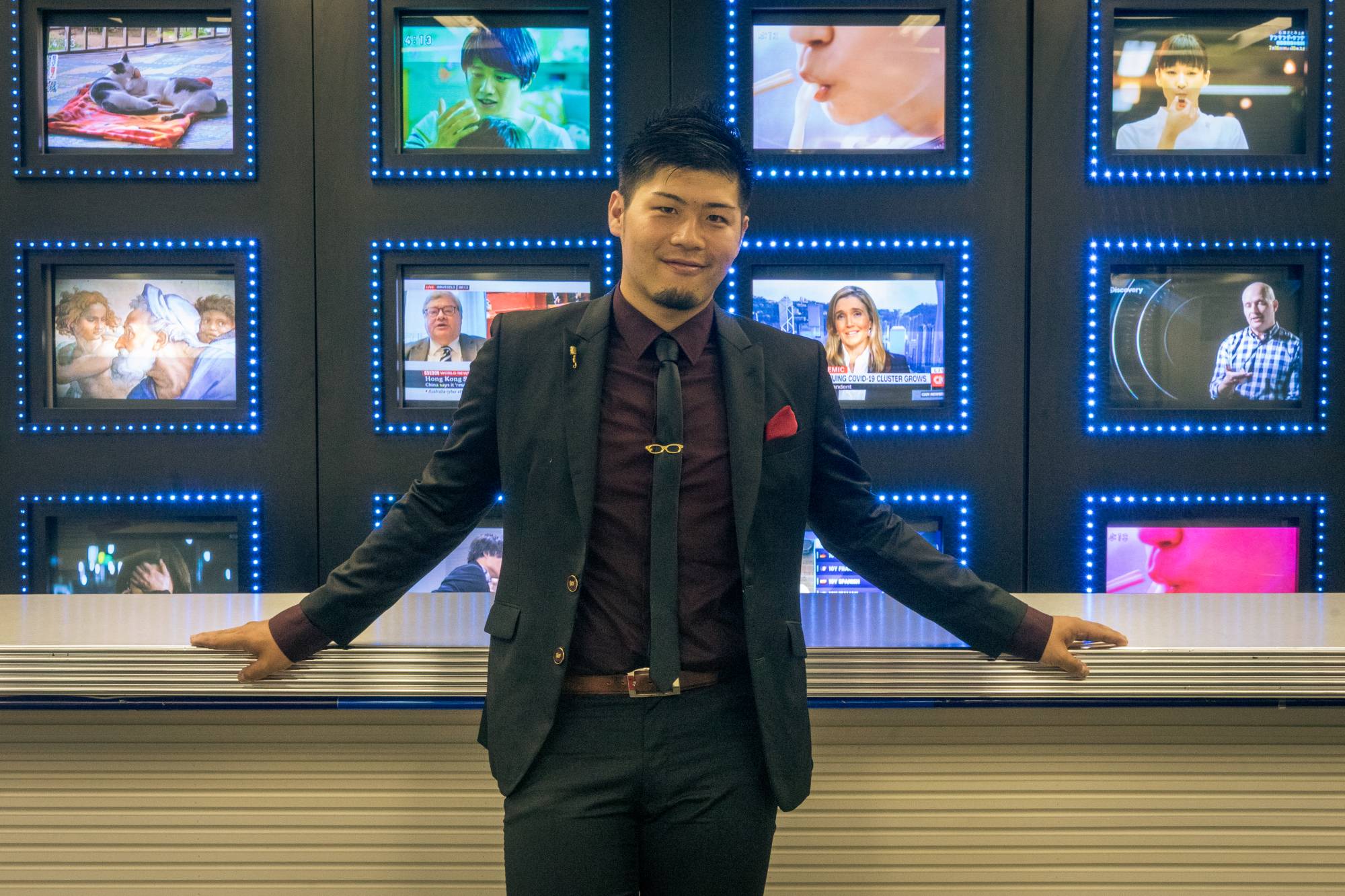In the photograph, an elegantly dressed Asian man stands confidently in front of a sleek chrome counter, leaning back slightly with his arms resting on the surface. He is adorned in a meticulously tailored black suit, complemented by a dark red shirt and a neatly folded red handkerchief in his left jacket pocket. The ensemble is accentuated with a stylish gold tie clip, resembling a pair of sunglasses, securing his thin black tie. His appearance is polished further with a brown belt and a well-groomed black goatee, and his hair is carefully styled, giving him a sophisticated look.

Behind him, a striking array of 12 small monitors, each encased in blue and white LED lights, displays a variety of channels. The screens showcase a diverse mix of content, including news programs, a racing event, a soap opera, a cooking show, and even a cat video. This eclectic mix suggests the setting might be a vibrant media entertainment area, possibly within a casino or a high-tech store. The man’s demeanor, combined with his stylish attire, gives the impression that he could either be an employee proud of his workplace or an individual enthusiastically showcasing his sophisticated look in this dynamic environment.